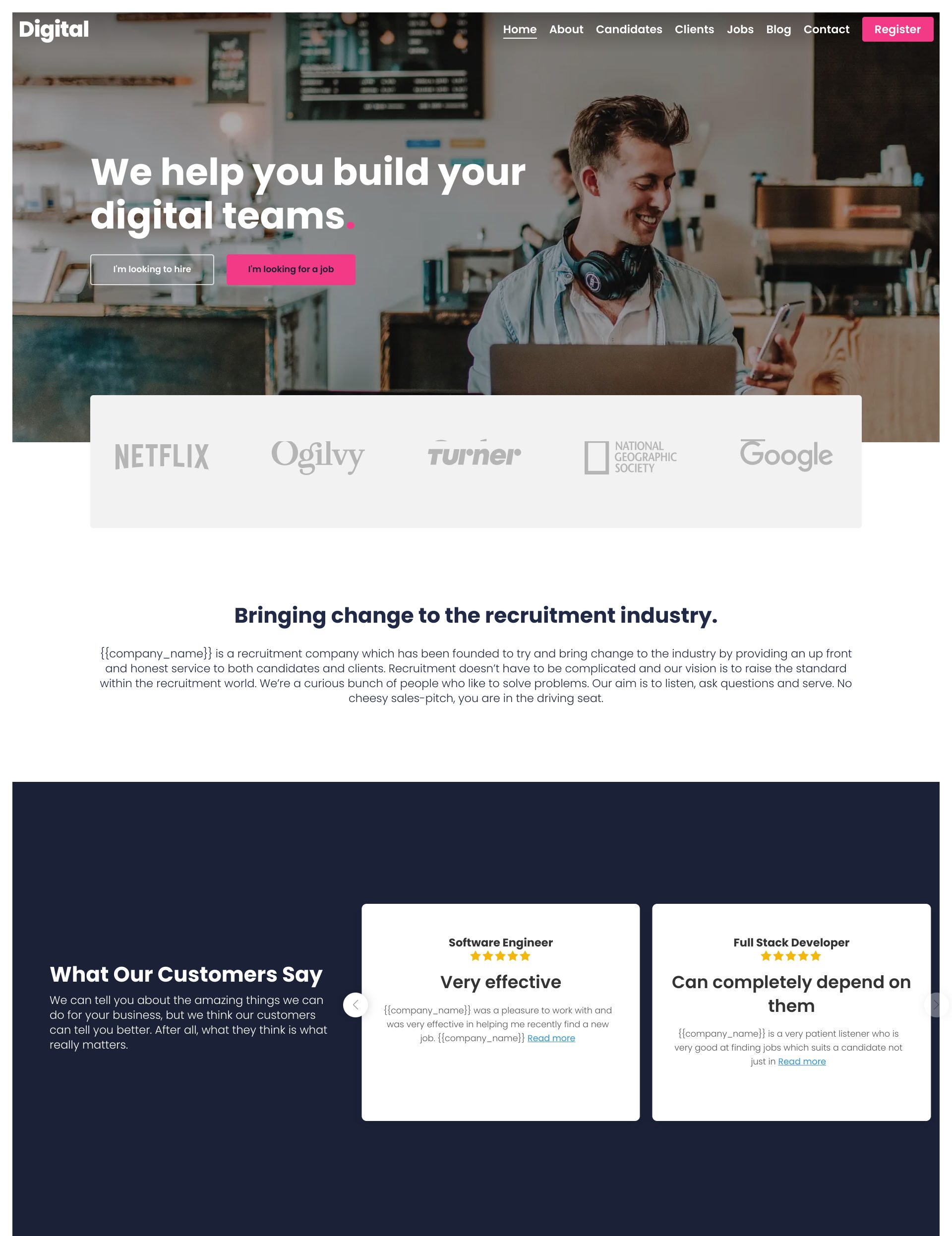The image showcases a website prominently titled "Digital" in the top left-hand corner. Central to the design is a large photograph of a young man donning headphones, engaged with both a smartphone and a laptop. Adjacent to this image on the left side, a conspicuous banner reads, “We help you build digital teams.” Beneath this banner are two buttons: one transparent button labeled "I'm looking to hire" and a pink button labeled "I'm looking for a job."

At the top of the screen, spanning from the center to the right, is a navigation bar featuring multiple menu options, including Home, About, Candidates, Clients, Jobs, Blog, Contact, and Register—the latter represented by a pink button.

Below the main image are logos of renowned companies such as Netflix, Ogilvy, Turner, National Geographic Society, and Google. This section is followed by a headline that declares, “Bringing change to the recruitment industry,” with accompanying text elaborating on the concept. At the bottom of the image, a dark blue rectangle features customer testimonials, including quotes from a software engineer and a full-stack developer, adding personal endorsements to the site's credibility and functionality.